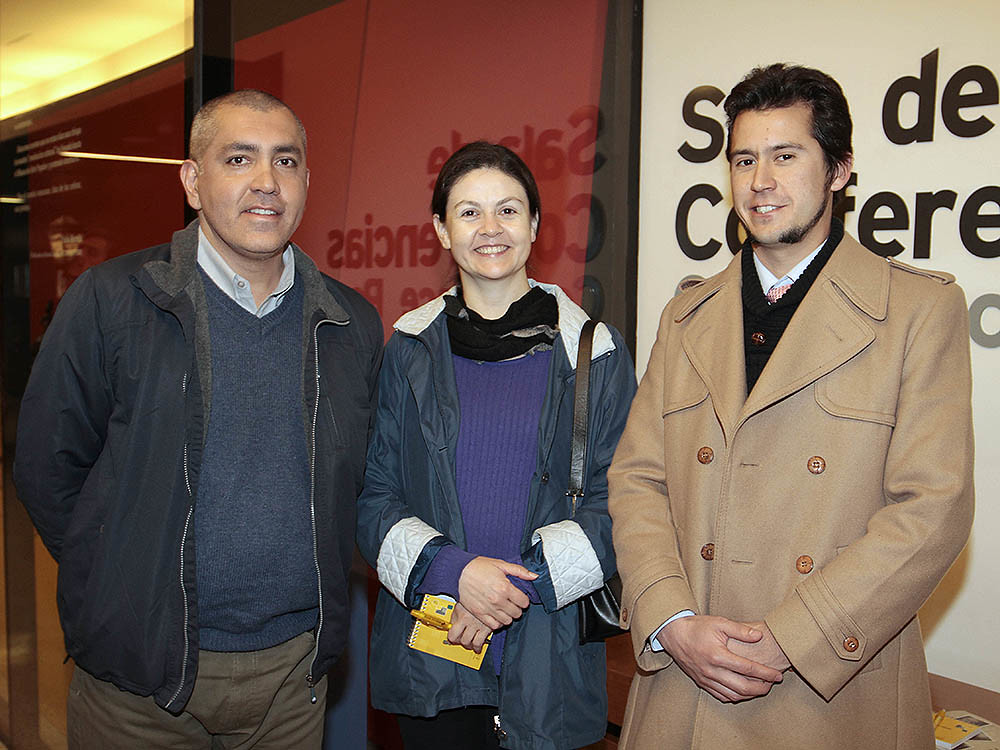In this photograph, three individuals stand together inside what appears to be a conference hall. The woman in the middle, who is smiling, has short brown hair and is wearing a blue jacket over a purple sweater. Her hands are crossed, holding a yellow notepad and pen. She also has a purse over her left shoulder. To her left is a man with a shaved head and in his 50s, dressed in a blue jacket, blue cardigan, and a light blue shirt, paired with gray pants. On her right is a younger man, likely in his 30s, wearing a beige trench coat, black vest, and collared shirt. He has short brown hair with noticeable sideburns. The background features a red and white wall with partially obscured lettering, suggesting it might be a section of a conference or exhibition space. The setting is illuminated, with a ceiling light casting a warm glow over the group.